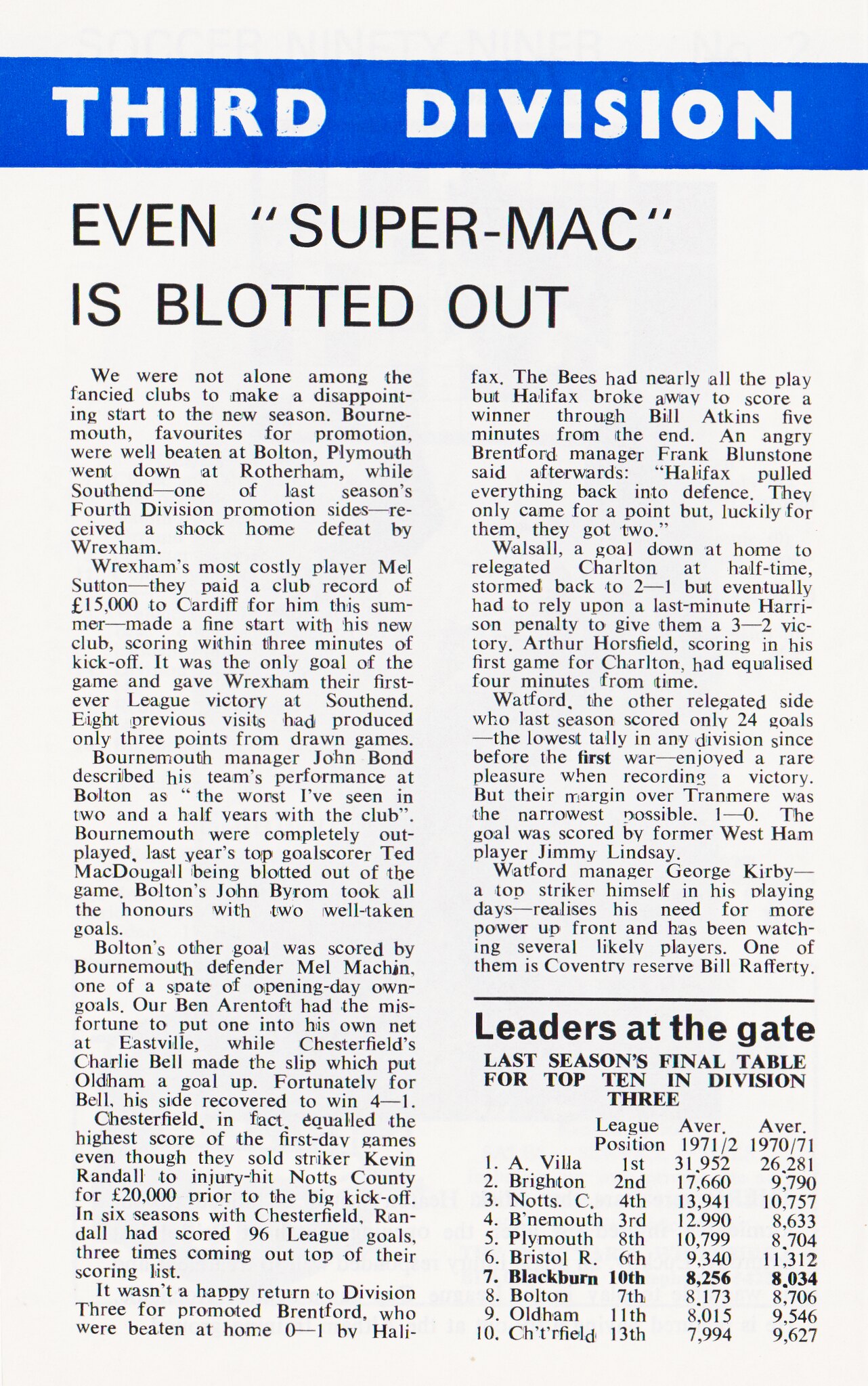The image shows a detailed newspaper article clip with a light green background, featuring a blue horizontal banner at the top with "THIRD DIVISION" written in bold white capital letters. Below the banner is the subheading, "Even Super Mac is Blotted Out," also stylized with quotation marks around "Super Mac." The article starts prominently from the top left and covers the recent beginning of a soccer season in the early 1970s. It discusses various teams' performances, including Bournemouth, Plymouth, Southend, West Ham, and more. Key highlights include player transfers, match outcomes, and specific anecdotes such as Wrexham's historic league victory at Southend, Bournemouth manager John Bond's critical remarks on his team's play, and Chesterfield's recovery to win after an own goal gaffe. At the bottom right of the article, a chart titled "Leaders at the Gate" lists the top ten Division III teams from the previous season (1971-72) along with their league positions and average attendance figures for the years 1971-72 and 1970-71. Notable entries include team A Wheeler with the highest attendance and Bolton mentioned for their significant performance changes. The piece is dense with statistical information and narrative details about the teams and their standings.